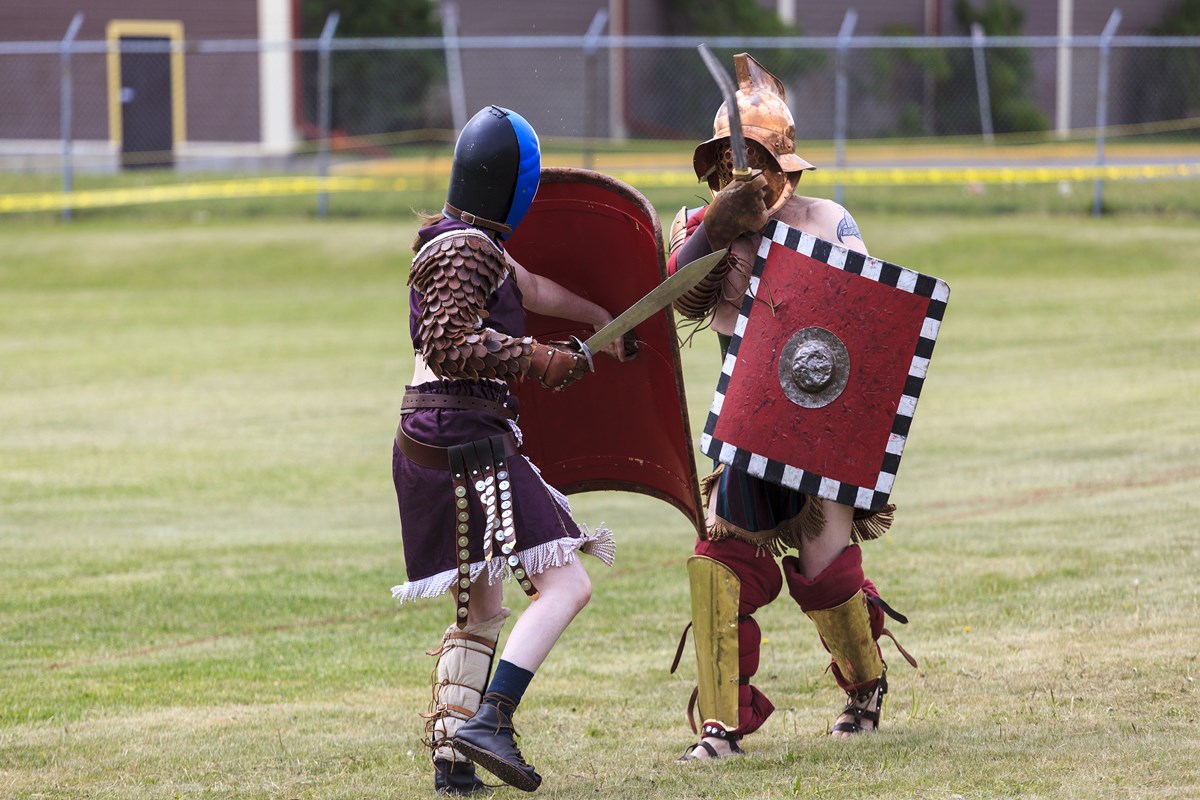In the image, two men are engaged in an intense sword fight on a grassy field. The terrain is a mix of light brown and green patches, possibly indicative of a school field or park, with a chain-link fence and blurred buildings in the background.

The man on the left, viewed from the back, wears a half-black, half-blue helmet, a piece of red armor on his chest, a black skirt that resembles a kilt, and black boots. He holds his sword to the right, set for an attack.

Opposing him, the man on the right, seen from the front, sports a yellow general-like hat, a mixture of yellow and red boots, and no shirt, showcasing a tattooed arm. He wields a shield with black and white edges in his right hand and a bent sword in his left. His attire includes makeshift leather pieces and possible cricket pads for shin guards, giving him a rough, assembled look.

Their battle, reminiscent of a medieval jousting tournament but far more primitive, is taking place under clear skies with scattered trees in the background, lending a casual yet dramatic atmosphere to the scene.